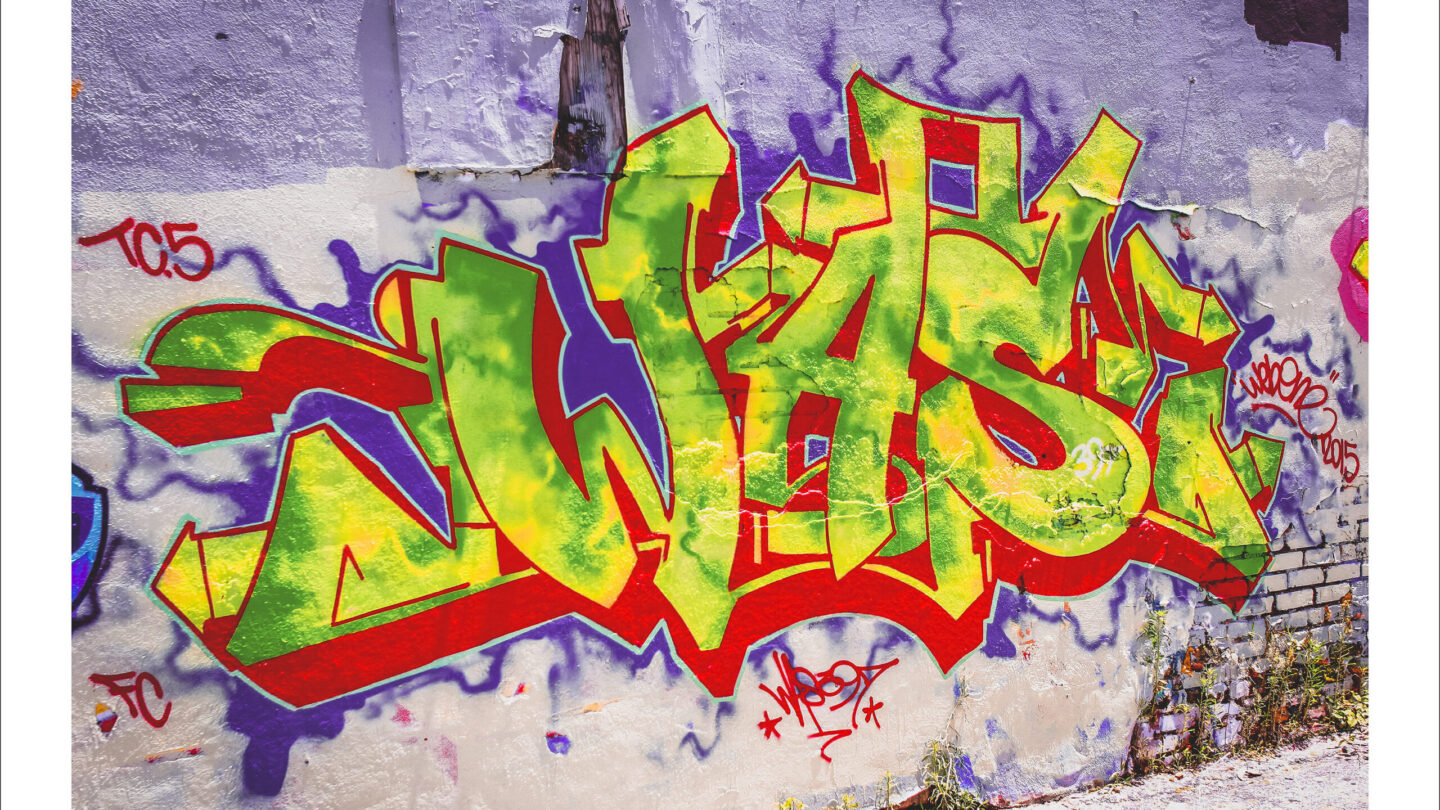The photograph captures a large brick wall dominated by vibrant graffiti. The wall itself is primarily painted over in a light lavender and white color, with some exposed white bricks visible at the bottom right. The graffiti includes a mix of bold colors—green, yellow, red, and purple—with additional highlights of light blue. Centrally, the graffiti appears to spell out "W.A.S." in green and yellow, surrounded by a complex mixture of red and purple borders. Additionally, there are red inscriptions that read "T-O.5" and "FC." Despite some difficulty in deciphering the exact text, the colorful mural stands out vividly against the relatively muted background. The image is horizontal and rectangular, accentuating the expansive nature of the wall and its intricate artwork.